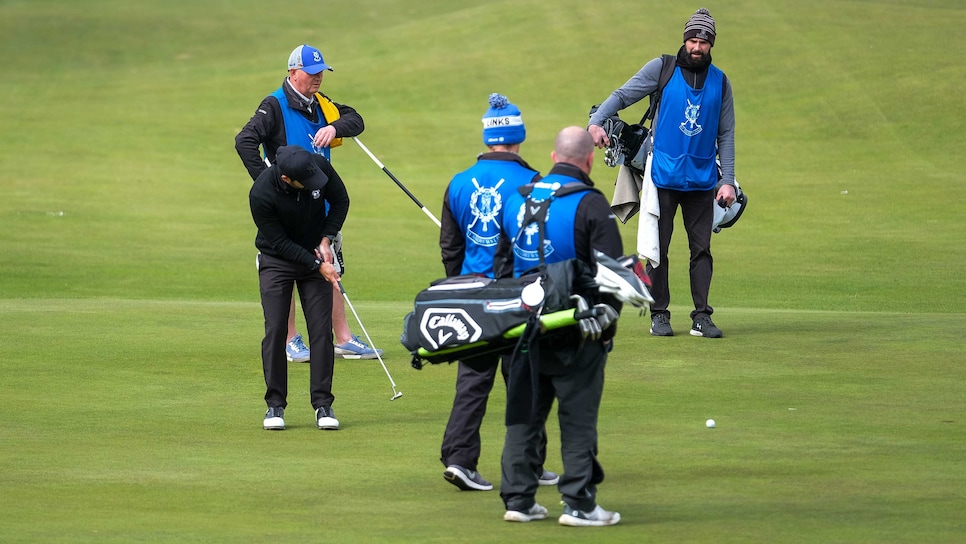In this detailed outdoor photograph taken at the historic St. Andrews Golf Course in Scotland, five men are positioned on the green, surrounded by the lush, velvety grass of the golf course. Central to the image is a golfer in mid-stroke, dressed entirely in black—including a long-sleeved shirt, trousers, and saddle shoes. The golfer, who wears a black baseball cap, is focused as he putts the ball towards the hole, which appears on the far right edge of the photo. 

Encircling the golfer are four caddies, all clad in bright blue vests emblazoned with the emblem and name "St. Andrews" on both the front and back. Two of the caddies stand behind the golfer, one holding a flagstick over his shoulder and the other carrying a golf bag. One of these caddies wears a blue knit cap, while the other is bald. On the far left, another caddy, distinct in his blue-gray baseball cap, is dressed in shorts, a black long-sleeved shirt, and black shoes. The remaining two caddies, each with a golf bag slung over their shoulders, are dressed in similar blue vests with black long-sleeved shirts and trousers. One of them, positioned on the far right, sports a long black beard and a blue knit cap.

The vibrant, meticulously manicured green of St. Andrews provides a scenic backdrop, highlighting the focused interaction between the single golfer and his attentive caddies. This image captures a moment of quiet concentration and teamwork at one of the most iconic venues in the golfing world.